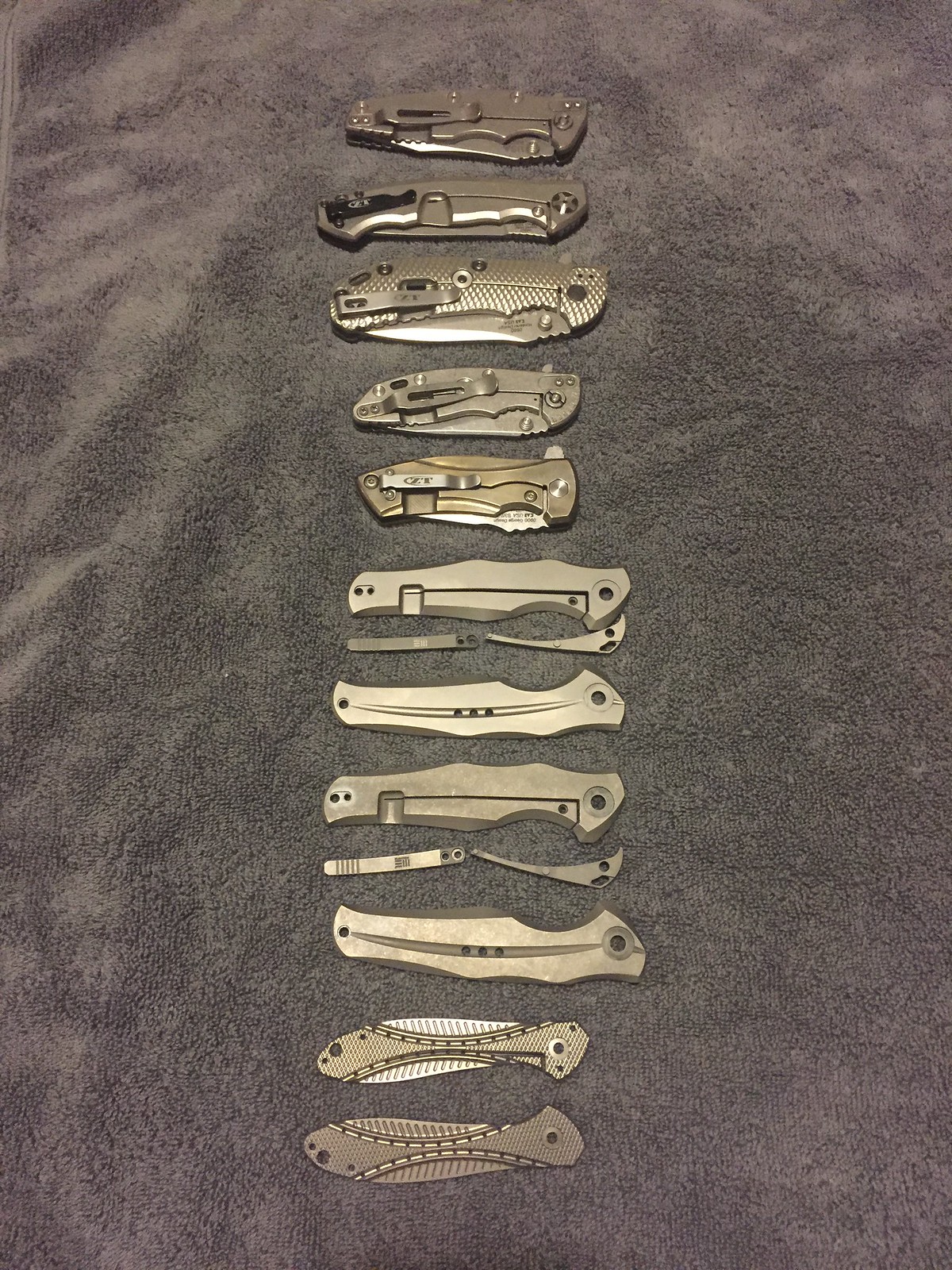This indoor, color photograph captures around a dozen folding knives meticulously displayed on a gray blanket. Arranged in a single column from top to bottom, all the knives are oriented horizontally with a silver or granite-like finish. At the top of this aligned collection, there is a multifunctional utility knife, reminiscent of a Swiss Army knife, featuring multiple tools that can be extended. The knives primarily feature plain silver designs, however, the third knife stands out with a textured crosshatch body. Further down, the bottom two knives exhibit distinctive stitching designs and oblique grooves on their blades. Notably, two knives have been disassembled, with their casing halves and blade attachments neatly laid out on the blanket. These disassembled knives seem to be models of the same type, adding an intriguing element to the orderly arrangement.